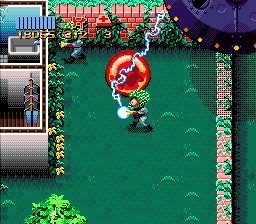This is a screenshot from an old video game, reminiscent of graphics from the 1980s or 1990s. The scene depicts a small, square-shaped area characterized by its pixelated art style. Central to the image is a little alien character with a large green head, pointy ears, and a striking red and white eye. The alien, dressed in a gray suit, appears to be charging a blue lightning bolt attack. Around its head is a glowing reddish-orange orb with a darker center.

The setting is a backyard area, with green grass surrounding a brown brick wall topped with foliage. Behind the character, in the top-right corner, there's a hovering UFO. The top of the screen shows a light gray building in a top-down view, exposing its interior with details such as clothing, plants, and what appears to be a bathtub and kitchen sink.

At the top left of the screen, there's a score displayed in golden numerals, "18055", followed by "312" and the digit "3" in orange. Directly below the score is a blue status bar, represented by a line of vertical light blue bars, likely indicating health or power levels. Additionally, the scene includes a plot of land with planted greenery alongside a green plant situated in the bottom-left corner of the yard.